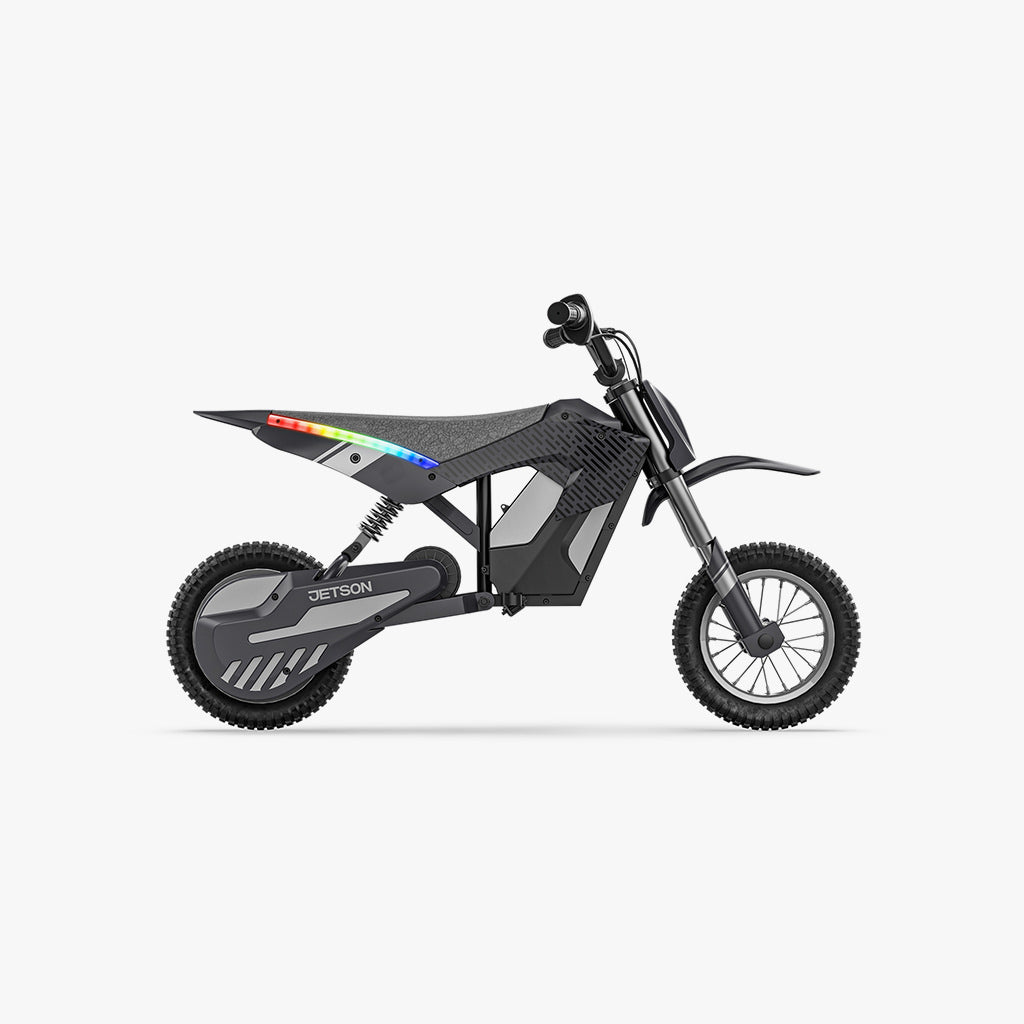This digital art rendering showcases a futuristic moped named Jetson, positioned against a blank white background. The moped is primarily constructed from various shades of dark and light gray panels. Its design features a distinctive spiky seat and a prominent, elevated front fender that appears almost separate from the rest of the bike except for a central connecting bar. A notable visual element is the rainbow-colored strip along the side, potentially representing illuminated RGB lighting, which transitions smoothly through multiple colors. The bike's frame resembles the shape of a '7,' with the front and rear wheels independently attached. The rear wheel is labeled "Detson," presumably indicating the brand. Additionally, the bike includes a spring mechanism near the rear wheel and delicate wire features leading to the front. Beneath the moped, a subtle shadow enhances the three-dimensional effect.